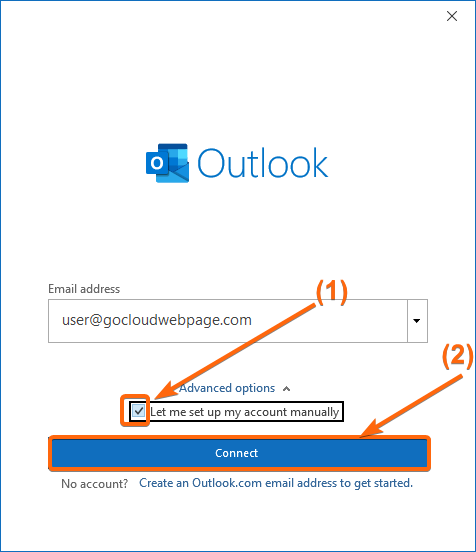The image is a color screenshot in portrait format showing the initial setup window for Microsoft Outlook. The top portion of the window displays the blue Outlook logo against a white background. Below the logo, there is a prompt to insert an email address, pre-filled with "user@gocloudwebpage.com". Adjacent to this, a blue hyperlink labeled "Advanced options" is available for those who want additional setup choices. The user has opted to tick the checkbox labeled "Let me set up my account manually". A large, prominent dark blue "Connect" button is situated directly beneath this checkbox. Below the "Connect" button, there's a prompt that reads, "No account? Create an outlook.com email address to get started."

Overlaying this screenshot are instructional annotations. An orange arrow labeled "1" points to the "Let me set up my account manually" checkbox, indicating the first step. A second orange arrow labeled "2" directs attention to the "Connect" button, highlighting it as the next step. These annotations appear to be guidance from a user or a tutorial intended to assist others with the setup process.